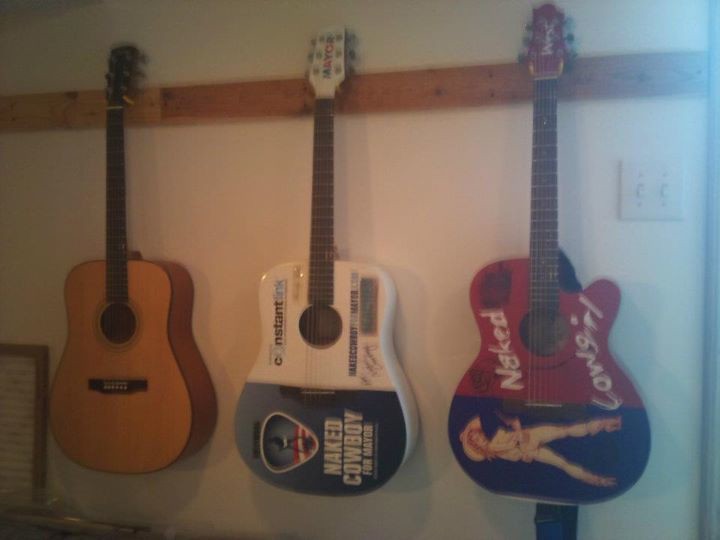The image depicts three guitars hanging on a horizontally mounted wooden plank on an off-white wall. The wooden plank, approximately the size of a one by six, features visible knots and variations in its wood grain and supports the guitars with pegs at their necks. The left guitar is a plain, standard acoustic guitar with a natural brown wooden body. The middle guitar is predominantly white with a bluish-gray bottom half, featuring the text "Naked Cowboy for Mayor" in white, accompanied by a triangle-shaped graphic and a cowboy design. On the right is an acoustic guitar with a red body and a darker bottom half, inscribed with "Naked Cowgirl" in white text; it showcases an illustrative design of a scantily clad cowgirl. The photo is slightly out-of-focus and poorly lit, adding a hazy effect, especially on the right side where a small light switch is visible.